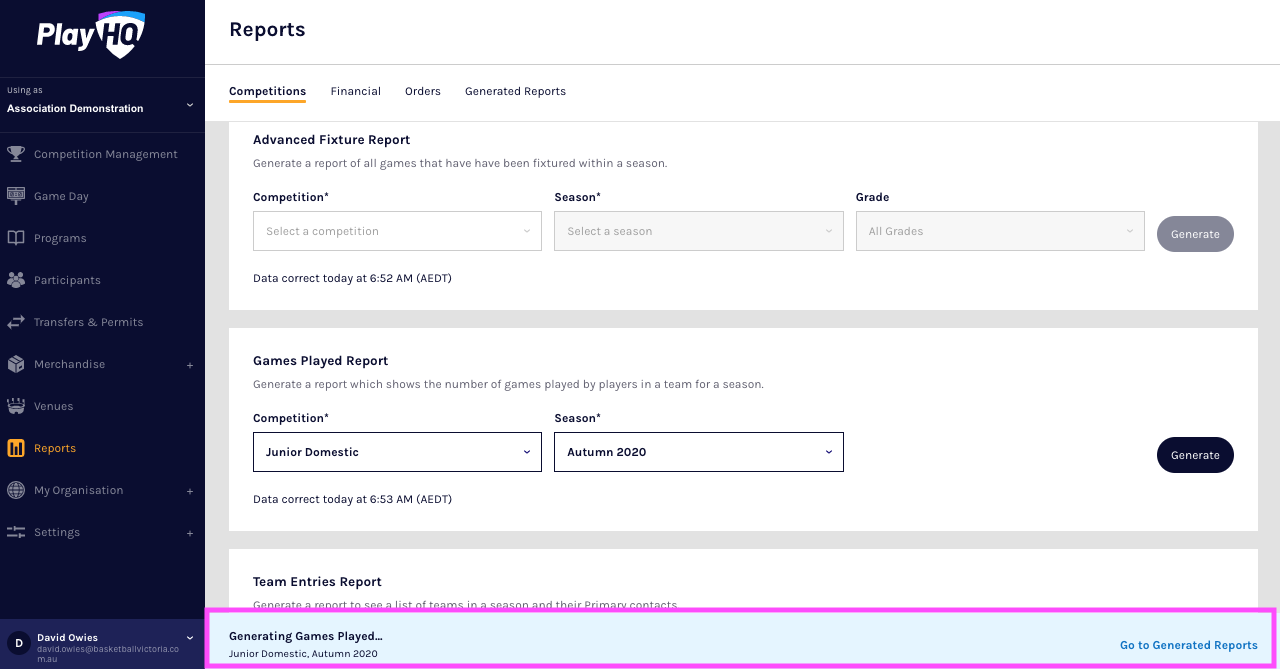Screenshot of PlayHQ Webpage Interface

This screenshot depicts the interface of a PlayHQ webpage, identified by the PlayHQ logo prominently displayed in the upper left corner. The left sidebar features a dark blue background, populated with light gray text and a few white-highlighted sections. From top to bottom, the sidebar lists various categories adorned with corresponding icons:

1. **Association Demonstration**: Text indicating the user's role or view.
2. **Competition Management**: Denoted by a trophy icon.
3. **Game Day**: Represented by a gaming controller icon.
4. **Programs**: Illustrated with a book icon.
5. **Participants**: Depicted with a people icon.
6. **Transfers and Permits**: Marked with a horizontal arrow icon.
7. **Merchandise**: Shown with a closed box icon.
8. **Venues**: Symbolized by an arena icon.
9. **Reports**: Highlighted in orange with a graph icon.
10. **My Organization**: Indicated by a globe icon.
11. **Settings**: Represented by a gear icon.

At the bottom of this sidebar, the logged-in user's name appears: "**David Owies**," displayed next to a profile icon featuring a white "D" on a black circle and a white dropdown arrow. Below the name, the associated email address is given: "**david.owies@basketballvictoria.com.au**."

The main section of the page, on the right, has a white background and is titled "**Reports**." Below this heading, options are listed as "**Competitions, Financial, Orders,**" and "**Generated Reports.**" An orange underline beneath "Competitions" indicates the current section being viewed.

In this section, multiple report options are presented, each within a white rectangular box:

1. **Advanced Figure Report**:
   - **Fixture Report**: A brief description states, "Generate a report of all games that have been fixtured within a season." It includes three dropdown fields labeled "Competition," "Season," and "Grade," and a gray circle button on the right labeled "Generate."

2. **Games Played Report**:
   - Description: "Generate a report which shows the number of games played by players in a team for a season."
   - Dropdown fields: "Competition" (currently set to "Junior Domestic") and "Season" (set to "Autumn 2020"), both of which are adjustable.
   - A timestamp showing "Data Correct Today at 6:53 AM (AEDT)."
   - A black elongated oval button with "Generate" in white text.

3. **Team Entries Report**:
   - Description: "Generate a report to see a list of teams in a season and their primary contacts." The full text is partially obscured by a purple-outlined horizontal rectangle containing the status message: "Generating Games Played, Junior Domestic, Autumn 2020" on the left, and "Go to Generated Reports" in blue hyperlink text on the right.

The right-most section of the page is cropped, but no additional text is visible beyond the categorized reports and options provided.

This detailed breakdown captures the essence of the PlayHQ interface in the presented screenshot, describing both visual elements and functional components clearly.